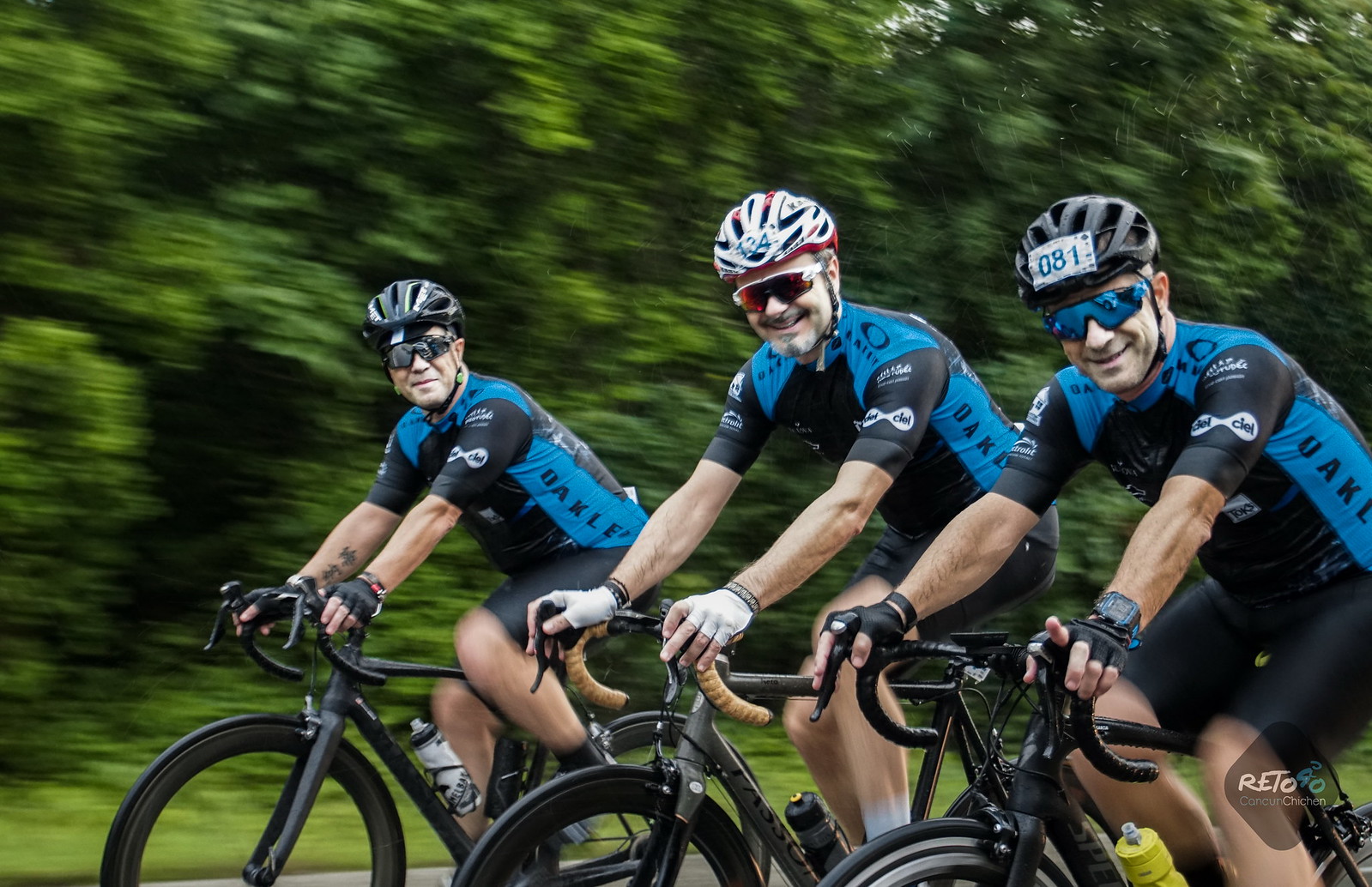The photograph captures a dynamic scene of three middle-aged Caucasian men cycling vigorously down a lush, wooded path, their spandex biking suits emblazoned with "Oakley," indicating a race or competitive event. The men are professional or semi-professional athletes, evident from their matching attire and numbered helmets (81, 134, and an obscured number), further signifying their participation in an organized race. The cyclists, all wearing different colored sunglasses and gloves, are captured in mid-motion, adding a strong sense of speed and energy to the image. They are smiling and looking directly at the camera as they pedal from the right-hand side towards the left, with the background blurred into a green haze of trees, emphasizing their swift passage through the wooded scenery. The scene is marked by the rich greenery of the trees and the grassy roadside. A subtle watermark reading "Reto, 40, Cancun, Xichang" is present in the right-hand corner of the photo.